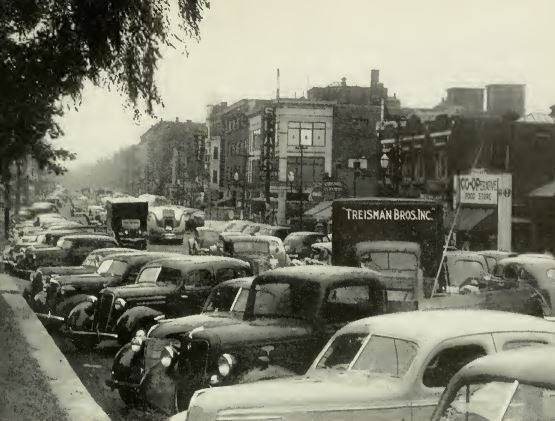The black-and-white photograph, likely taken in the 1930s or 1940s, captures a busy city or town street scene. The cars, with their rounded hoods, big grills, and large round lights, are parked perpendicularly to the sidewalks on both sides of the road. The street is lined with buildings, ranging from two to six stories, exhibiting the architectural styles of the early 20th century. In the middle of the street, a noticeable truck bearing the name "Treisman Brothers, Inc." stands out. The cloudy, sunless sky adds a subdued tone to the bustling atmosphere of the period, emphasizing the everyday hustle of this urban setting.